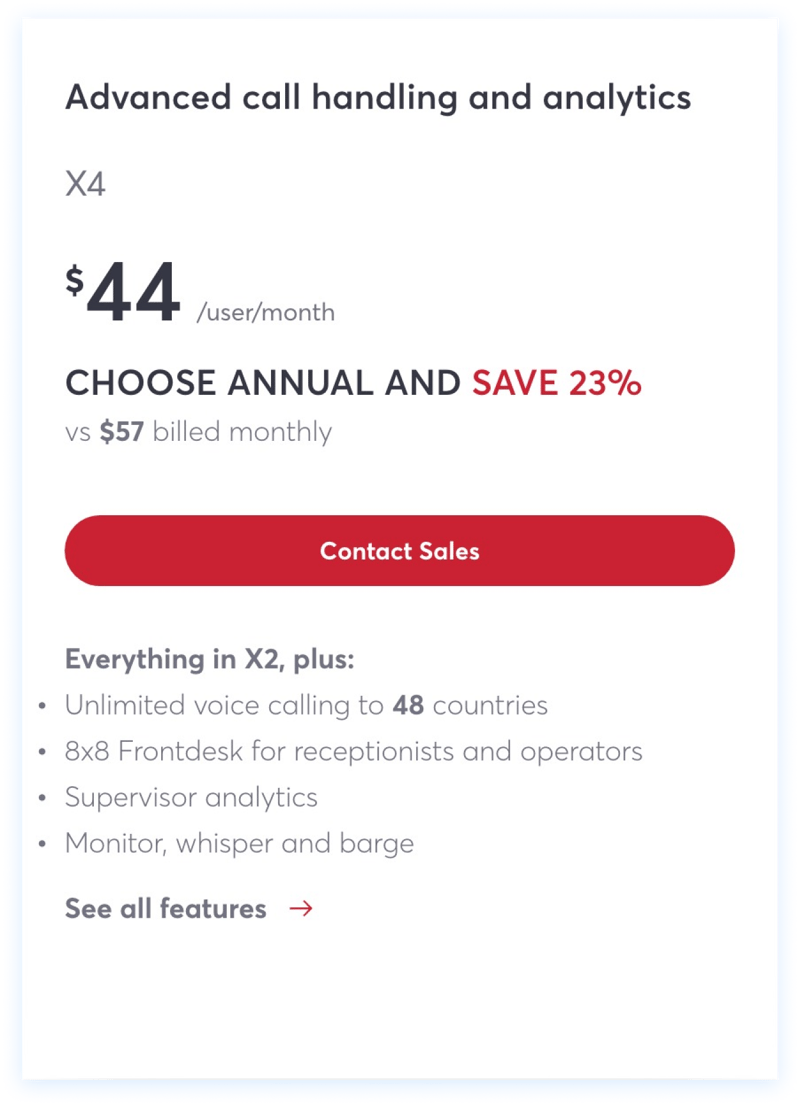The image is an advertisement highlighting advanced call handling and analytics features. At the top of the ad, the text "Advanced Call Handling and Analytics" is prominently displayed. Beneath this, in smaller gray font, is the label "X4." Further down, a small dollar sign is followed by the price "$44/user/month," where "$44" is in a larger font compared to the smaller gray "user/month" text. Next, the advertisement suggests opting for an annual plan to save 23%, versus a monthly billing rate of "$57." Below this pricing information, a large red button with the text “Contact Sales” in white font invites users to take action. Finally, the ad mentions that the X4 plan includes "everything in X2 plus" and lists four bullet points with additional features.